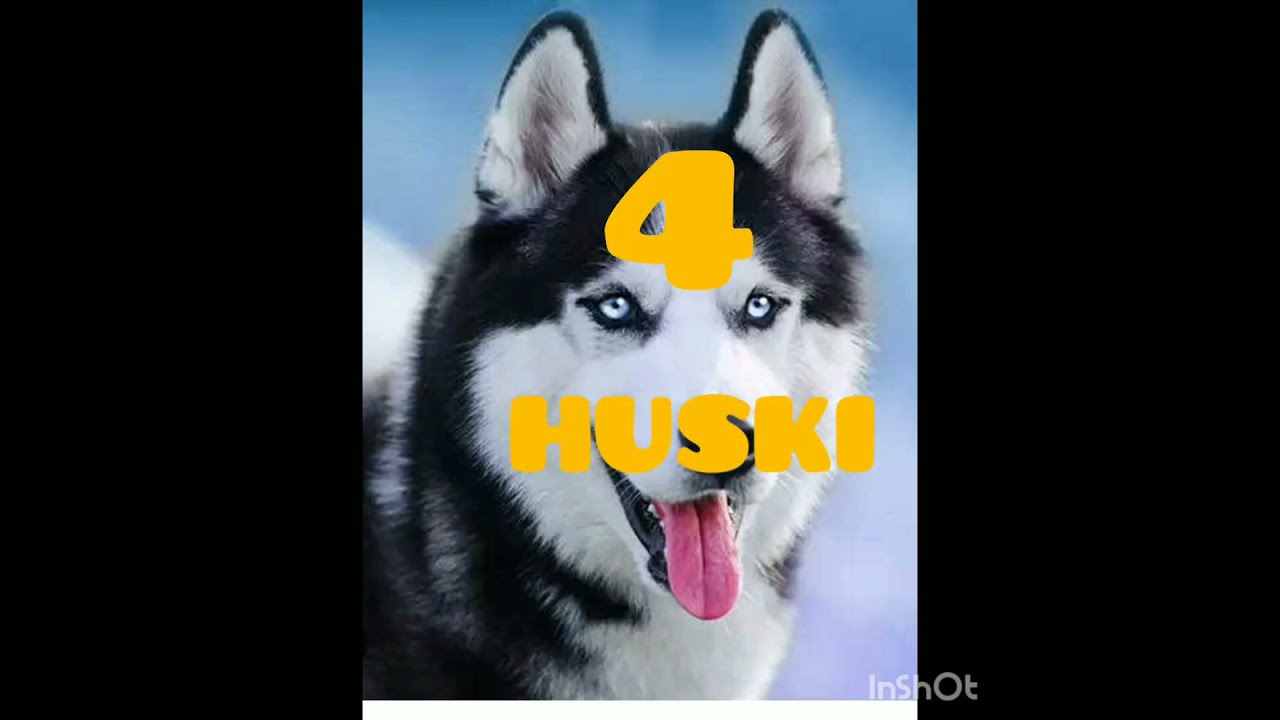The portrait-oriented photograph features a close-up of a striking black and white husky head, with its face filling the entire frame. The husky's brilliant turquoise-blue eyes gaze slightly to the right, and its pink tongue hangs out in a playful pant. The ears are perked straight up, showcasing the contrast between their dark exteriors and white interiors. At the top of the image, bold yellow font displays the number "4" above the misspelled word "huski." The bottom right corner contains a white "in shot" logo, likely a photo credit. The sides of the photo are framed with black bars, making the image fit within a landscape frame, and a clear blue sky can be seen in the background. Although the husky looks impressively realistic, some might mistake it for a well-crafted graphic due to its polished appearance.